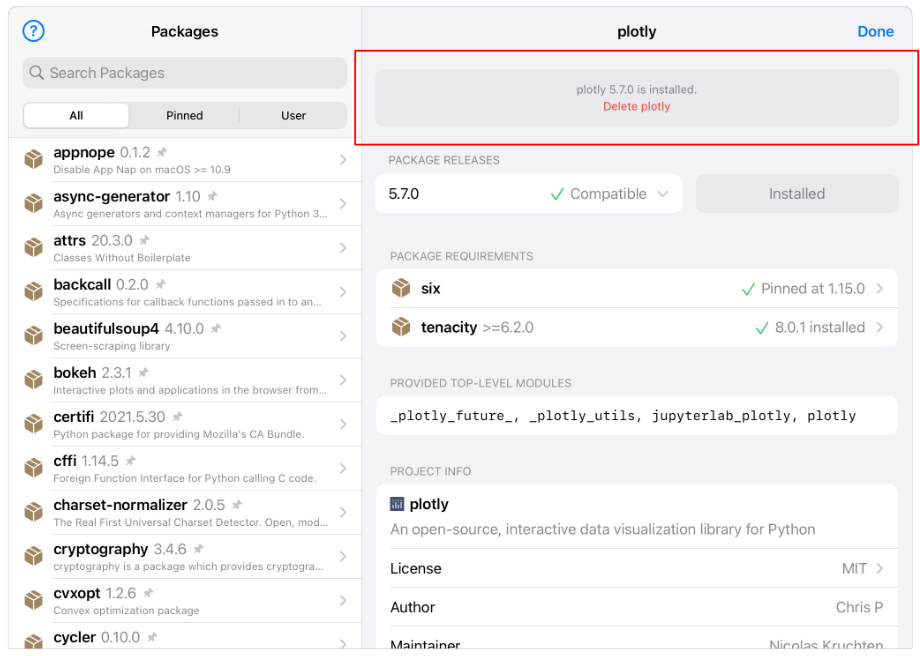The screenshot displays the package manager interface of a software development environment, highlighting the installation and management details of the Plotly library.

At the top, there are tabs labeled "Packages," "Plotly," and "Done," with a search bar labeled "Search Packages." Below, the page is divided into two columns. 

On the left column, there's a list of various installed packages including:
- AppNope 0.1.2: Disables AppNap on Mac OS 10.9.
- Async Generator 1.10
- ATTRS 20.3.0
- Batcall 0.2.0
- BeautifulSoup 4.10.0
- Boca 2.3.0
- Certify 2021.5.30
- CFFI 1.14.5
- CharzNormalizer 2.0.05
- Cryptography 3.4.6
- CVXOpt 1.2.6
- Cycler 0.10.0

The right column is focused on the Plotly package, specifically version 5.7.0, which is installed. This section shows:
- Release version: 5.7.0
- Compatibility and installation status: Compatible and Installed
- Package requirements: 6
- Pinned version: 1.15.0
- Additional modules and versions (e.g., Tenacity, Arrow at 6.2.0, Checkmark at 8.0.1)

There is a red box outlining the Plotly package, indicating an action such as "Delete." Additional annotations include:
- Plotly, an open-source interactive data visualization library for Python
- License: MIT
- Author: Chris P
- Maintainer: Nicholas Crutchton

Moreover, modules such as Plotly_utils, JupyterLab_Plotly, and others associated with Plotly are also mentioned, emphasizing its comprehensive integration with various tools.

This organized presentation helps users easily manage their packages and understand the dependencies and details of each package installed in their environment.